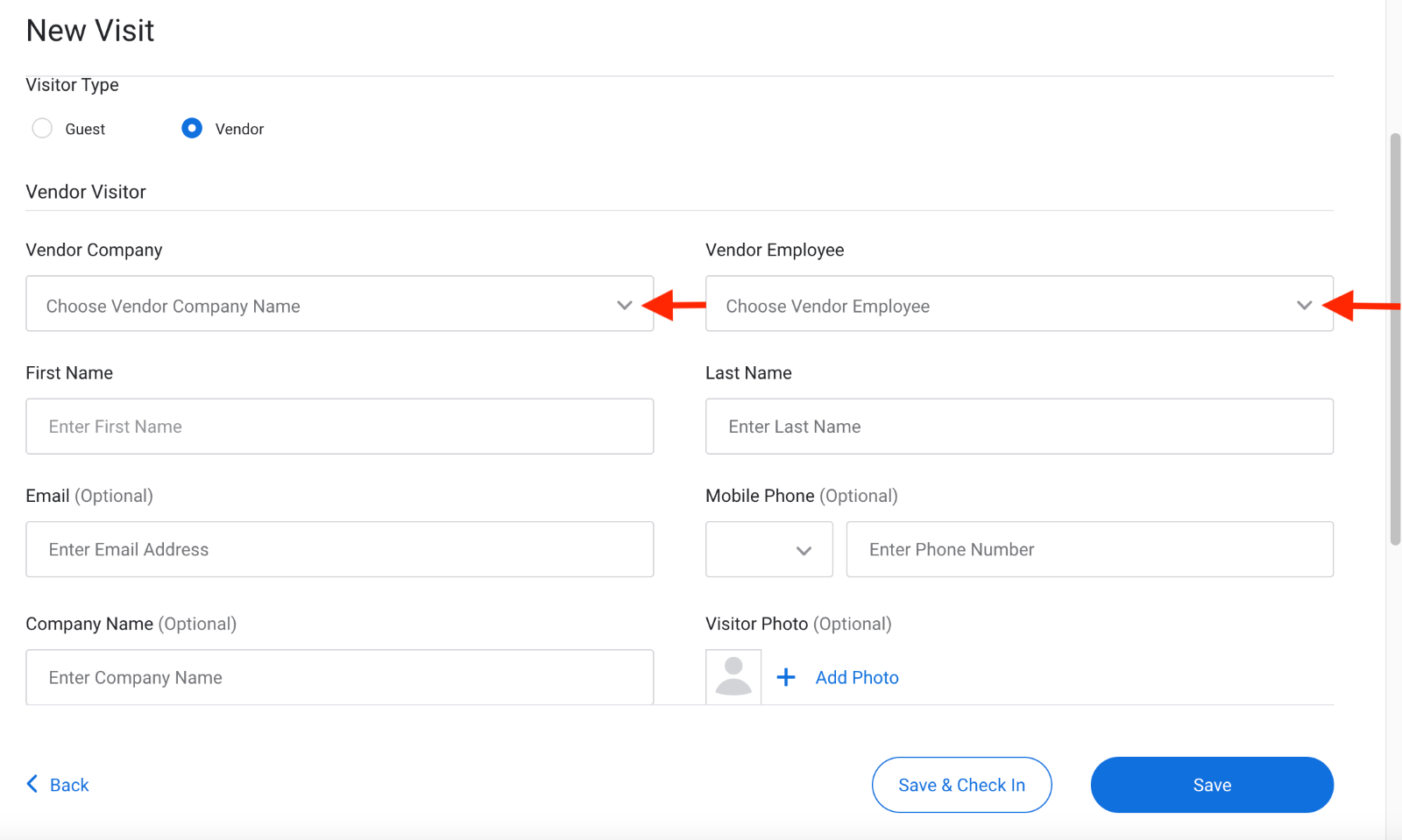The image displays a web page interface titled "New Visit" at the top left, designed for check-ins. The form comprises multiple fields tailored for different visitor types, with "Vendor" selected in this instance, triggering specific input requirements. The outlined sections include drop-down menus for "Vendor Company" and "Vendor Employee," mandatory fields for "First Name" and "Last Name," and optional fields for "Email," "Company Name," and "Mobile Number." Additionally, there's an "Add Photo" button adjacent to the "Visitor Photo" section, also optional. The interface features a white background with primarily black text and blue highlights. Red arrows have been edited into the image to emphasize the "Vendor Employee" and "Vendor Company" drop-downs. At the bottom, users can choose to "Save and Check-In" or simply "Save" using a blue button. The exact context of the check-in remains unclear, though it vaguely suggests a setting like a hospital.